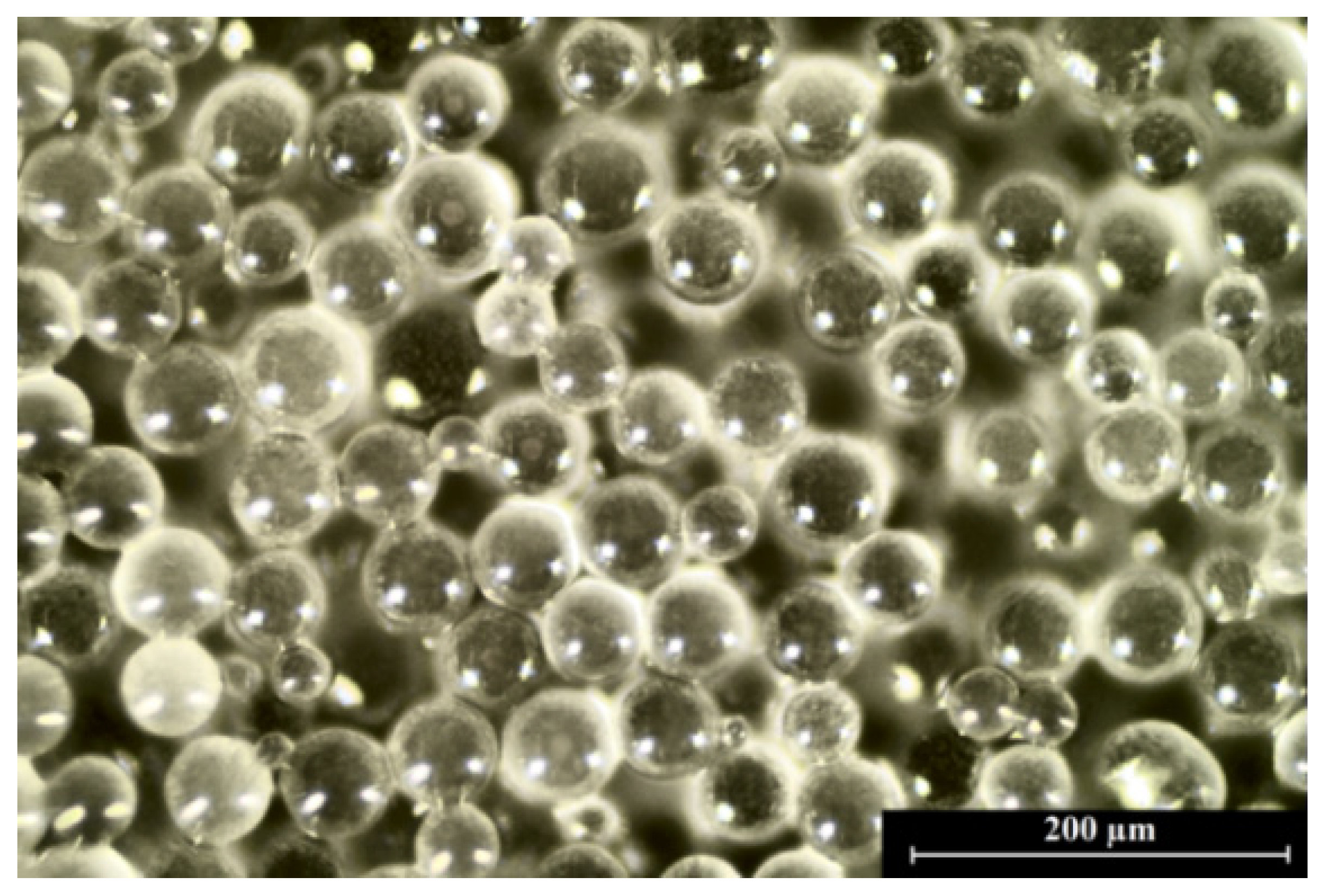This image appears to be a highly magnified view possibly taken with a microscope, showcasing a cluster of small, spherical, bubble-like structures. The bubbles, varying slightly in size but generally uniform, seem to be organized and layered together, suggesting they might be cells or microscopic organisms. The image has a dark background with light contrasts, giving a detailed and somewhat precise yet slightly grainy appearance. The colors are primarily green and white, with a wet-looking reflective quality that adds to the impression of a biological sample. In the bottom right corner, a black box features a scale indicating "200 micrometers," reinforcing the micro-scale nature of the photograph.